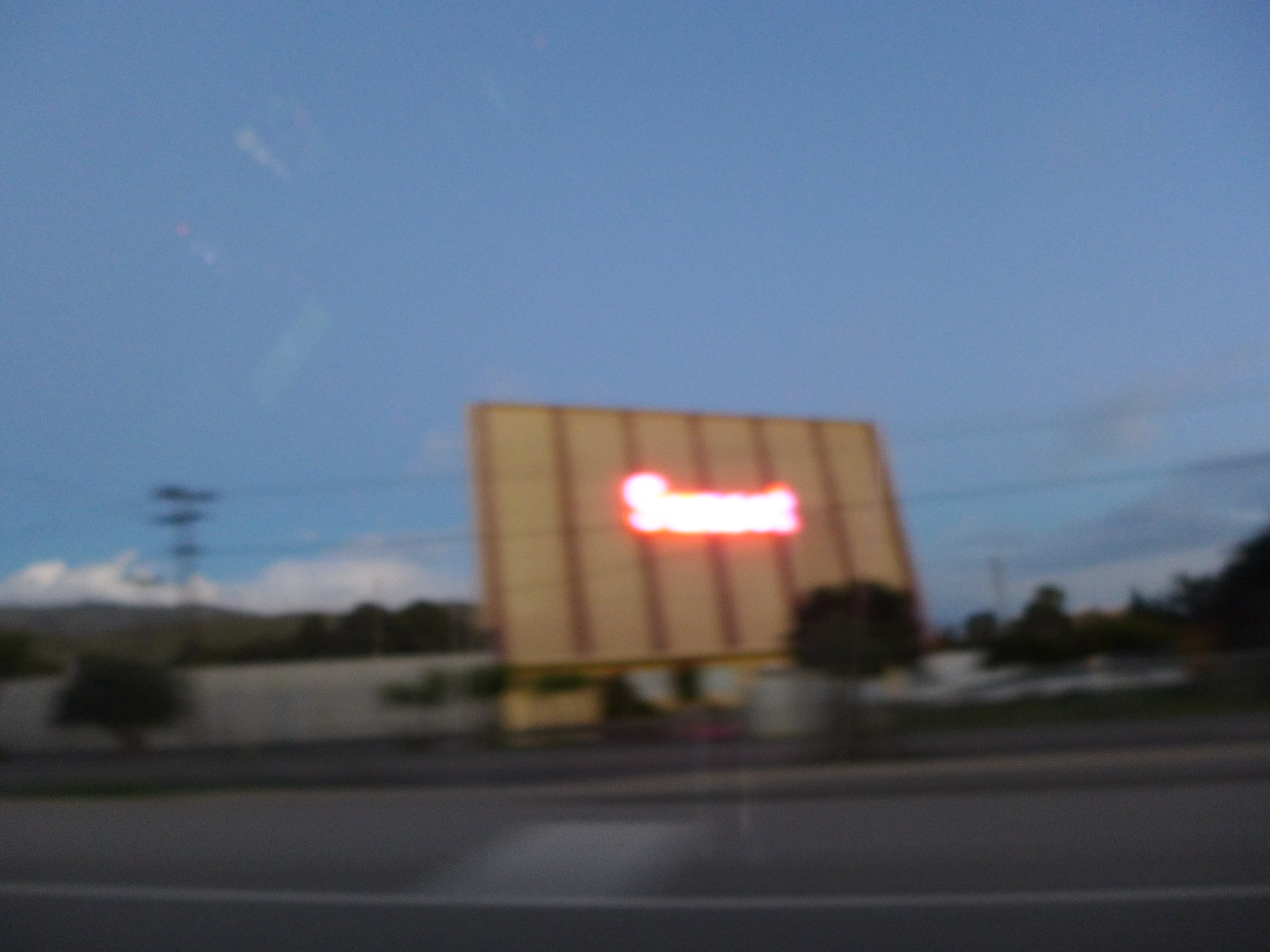A blurry, out-of-focus image captures an enigmatic scene under a dark blue evening sky. Spanning across the background are telegraph wires, adding a touch of urban complexity. Dominating the middle ground is a large hoarding, seemingly an advertisement billboard, illuminated by an unreadable neon sign. The billboard is notably split into six round sections, each separated by distinct stripes. In the foreground, silhouettes of trees and a stretch of highway hint at a bustling environment. The scene evokes curiosity, leaving viewers pondering the message behind the brightly lit, yet indecipherable, advertisement.